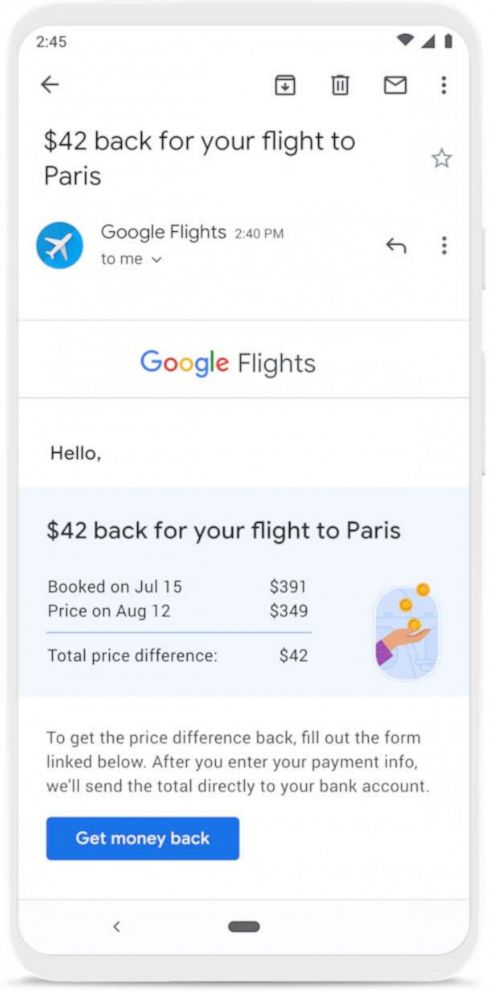In the screenshot of a smartphone, displaying a website, the current time in the top left corner reads 2:45, though it does not specify whether it is AM or PM. To the right of the time, the status bar icons indicate that the device has full Wi-Fi connectivity, maximum cellular signal bars, and a fully charged battery. On the screen, there are interactive buttons, including a back arrow for exiting, a download button, a trash can icon for deleting, an envelope icon for email, and a three-dot menu for additional options.

Below these icons, there is a message informing the user of a refund for their flight to Paris. The message is highlighted with a star symbol and features a blue icon with a white airplane, identified as a notification from Google Flights at 2:40 PM. The email header reads "Google Flights" and provides details about the refund: "Hello, $42 back for your flight to Paris." The booking date is listed as July 15th, with the price on August 12th showing a decrease from $391 to $349, resulting in a $42 price difference. The email instructs the user to complete a form via the included link to claim the refund.